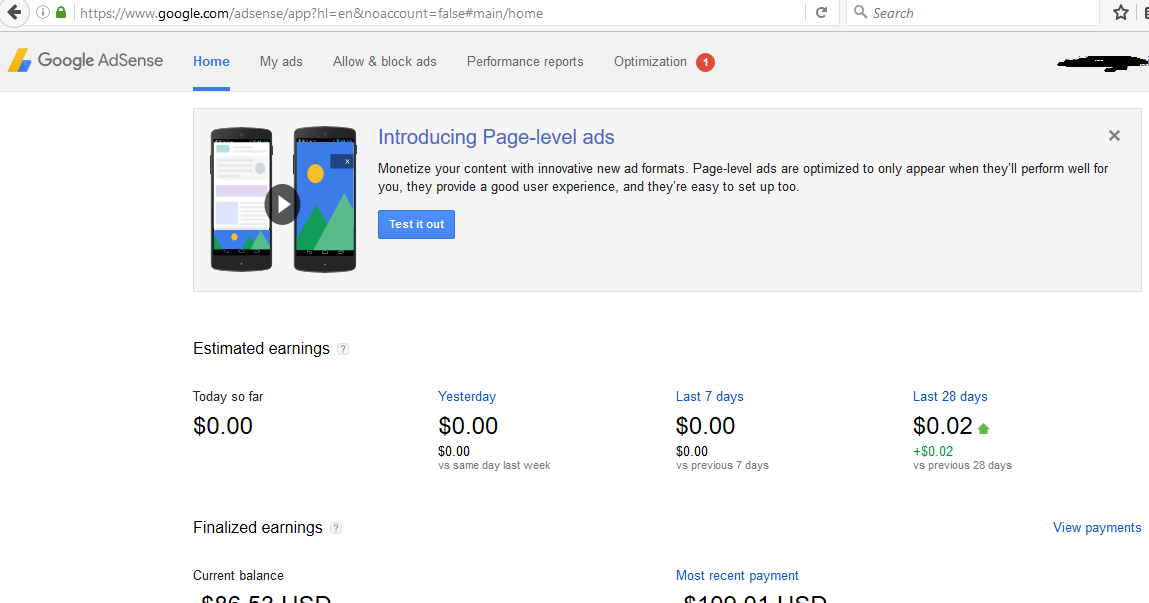The displayed image features a Google AdSense user interface. At the very top of the page is the URL address, accompanied by a search bar on the right. Beneath the header, labeled 'Google AdSense,' are navigational tabs: Home, Ads, Allow & Block Ads, Performance Reports, Optimization, with a notification marker indicating '1.'

On the far right, there is a section that has been manually blacked out, possibly obscured with a Sharpie, rendering its contents unreadable.

The central part of the display showcases an advertisement for Page Level Ads, with two types of cell phones depicted. The text reads, "Introducing Page Level Ads. Monetize your content with innovative new ad formats. Page level ads are optimized to only appear when they'll perform well for you. They provide a good user experience, and they're easy to set up too. Test it out."

Below the promotional content, there is a financial summary chart. The 'Estimated Earnings' section lists the following values: Today: $0.00, Yesterday: $0.00, Last 7 days: $0.00, Last 28 days: $0.02. The 'Finalized Earnings' section appears to be cut off and is not fully visible.